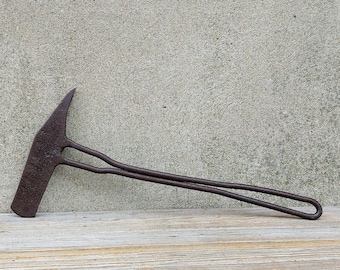This image shows a metal tool under construction on a light gray and tan wooden table, with a light and dark gray speckled wall behind it. The tool, potentially an unfinished hammer or axe, features a thin piece of dark chrome-colored metal. Its handle, made from two folded bits of metal wire, lies flat on the table. The rectangular tool head is flat on one end while the other end tapers into a sharp spike, giving it a dual functionality. The hammer-like tool appears forged, with its flattened head resembling an item squished by a heavy press.